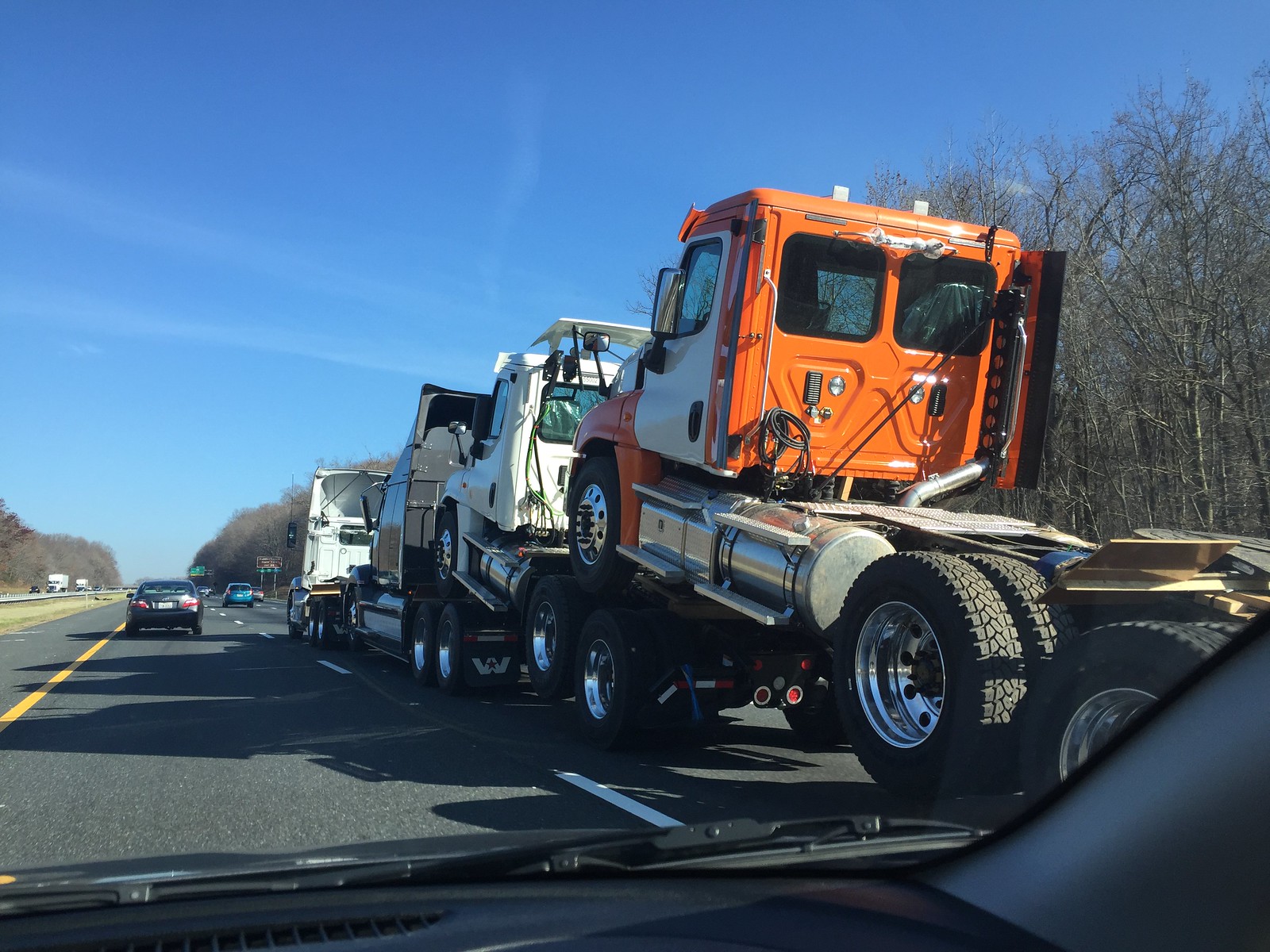The image is a color photograph taken from inside a vehicle, showing the view through the windshield with parts of the dashboard, windscreen wiper, and the right pillar visible. The scene is set on a highway with dark tarmac, marked by a yellow line on the left and intermittent white stripes down the center. In the distance to the right, the photograph prominently features a truck towing three semi-truck cabs stacked one behind the other. The leading truck is hauling the cabs, which are of differing colors: orange at the back, white in the middle, and black in the front. Further ahead, a dark car is visible on the road. Tall, leafless trees line the right side, suggesting either an early spring or winter setting under a clear, vividly blue sky streaked with horizontal white wisps, possibly clouds or airplane contrails.